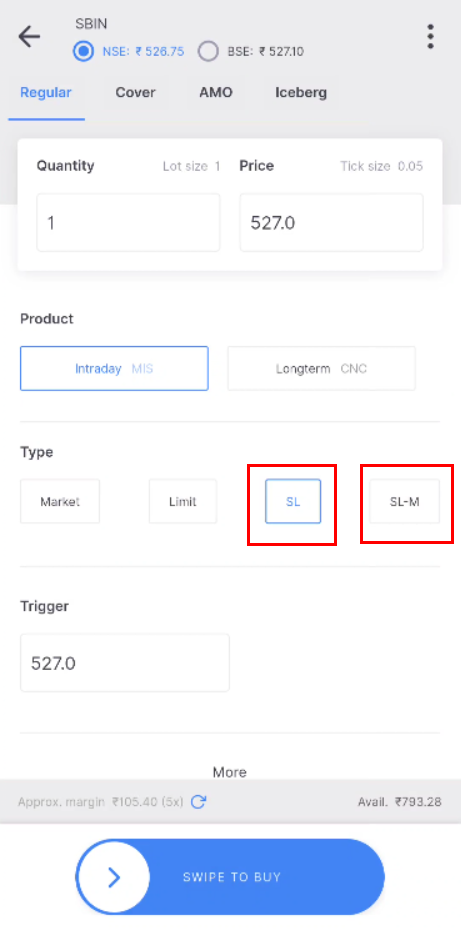The image depicts an intricate mobile application interface designed for stock trading. At the top of the screen, there are three standard buttons for additional information or options, commonly found in phone apps. Next to these buttons is a back arrow for navigation.

Prominently displayed at the top of the interface are stock details, including an identifier, "NAC," with a current value of 526.75 and a BSE listing of 527.10. Additional details include the quantity and price, presented as "1 @ 527." The tick size is specified as 0.05, while the lot size is 0.

Beneath these details are four navigation tabs labeled "Regular," "Cover," "AMO," and "Iceberg," indicating various trading options. The product type is marked as "Intraday MIS," with two selectable options below: "Intraday MIS" and "Long-term CNC."

Further down, there are four buttons labeled "Type," "Market," "Limit," "SL," and "SL-M," each representing different order types. Below these, a section titled "Trigger" includes a box for entering the trigger price, currently set at 527.0.

The interface also displays an "Approximate Margin" with a dynamic refresh feature, showing an available balance of $793.28. At the bottom of the screen, there is a prominent "Swipe to Buy" button for executing the trade.